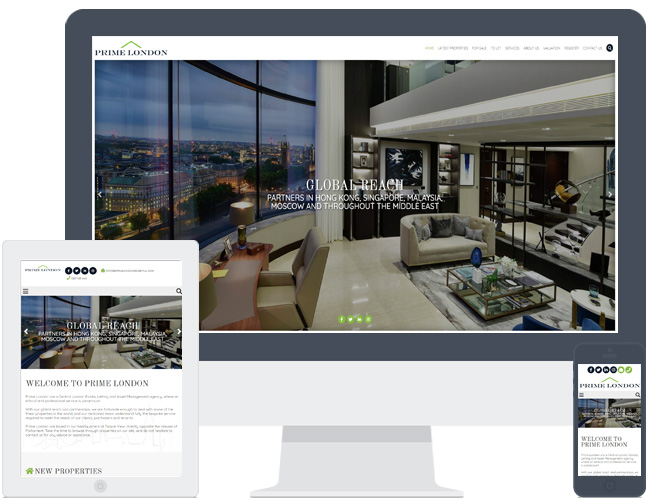A high-resolution image displays a computer monitor at the center, with a tablet positioned at the bottom left and a smartphone at the bottom right. The screen on the computer monitor showcases a website for "Prime London" with a green triangle logo above the text. The primary image on the monitor depicts a luxurious hotel or apartment suite, featuring a large window that offers a breathtaking view of the city at night. In front of the window sits a desk, accompanied by a chair and couch, creating a sophisticated, cosmopolitan atmosphere. The right wall appears lined with mirrors, enhancing the room's spacious and elegant design. 

Prominently centered on the screen is the text "Global Reach Partners in Hong Kong, Singapore, Malaysia, Moscow, and throughout the Middle East," highlighting the company's extensive international presence.

The tablet, with a sleek silver-white exterior, shows the same image of the elegantly furnished room, beneath which appear the words "Welcome to Prime London" followed by additional text. On the black smartphone to the right, the same room image is displayed, emphasizing the seamless access to Prime London’s information across multiple devices. This image effectively communicates the accessibility of Prime London’s services via computer, tablet, or mobile phone, underscoring the brand's commitment to user convenience and reach.